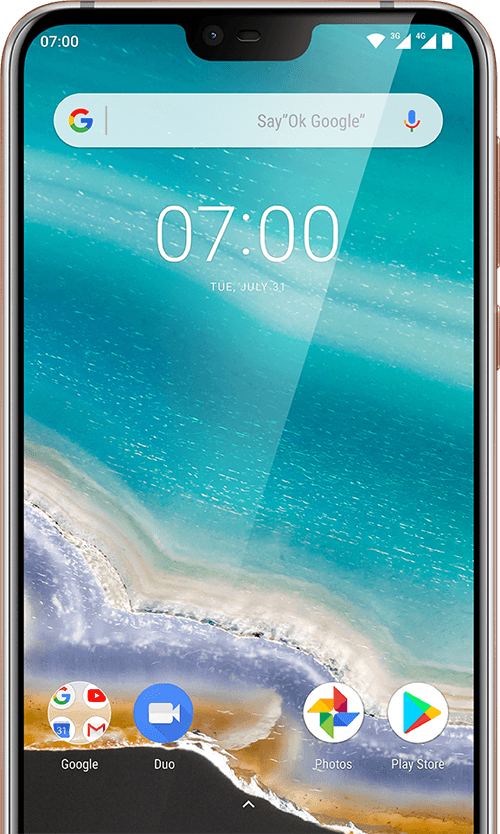A cropped screenshot of a Google phone's front page showcases a striking background resembling a piece of acrylic art painted to emulate the ocean. Dominating the top of the screen is an expansive search bar featuring the Google 'G' logo on the left. Adjacent to it, gray text prompts users with "Say, OK Google," followed by a microphone icon for voice searches. Centrally positioned on the screen is the time display, reading "07:00," accompanied by the date, "Tuesday, July 21st." 

At the screen's bottom, four icons are neatly arranged. On the far left, a circular folder labeled "Google" encloses icons for Google, YouTube, Google Docs, and Gmail. Next to it is the camera icon. Skipping a space in the middle, the Google Photos icon appears, followed by the Play Store icon on the far right. The phone's bottom edge is cropped out of the image, adding a sense of focus to the upper elements.